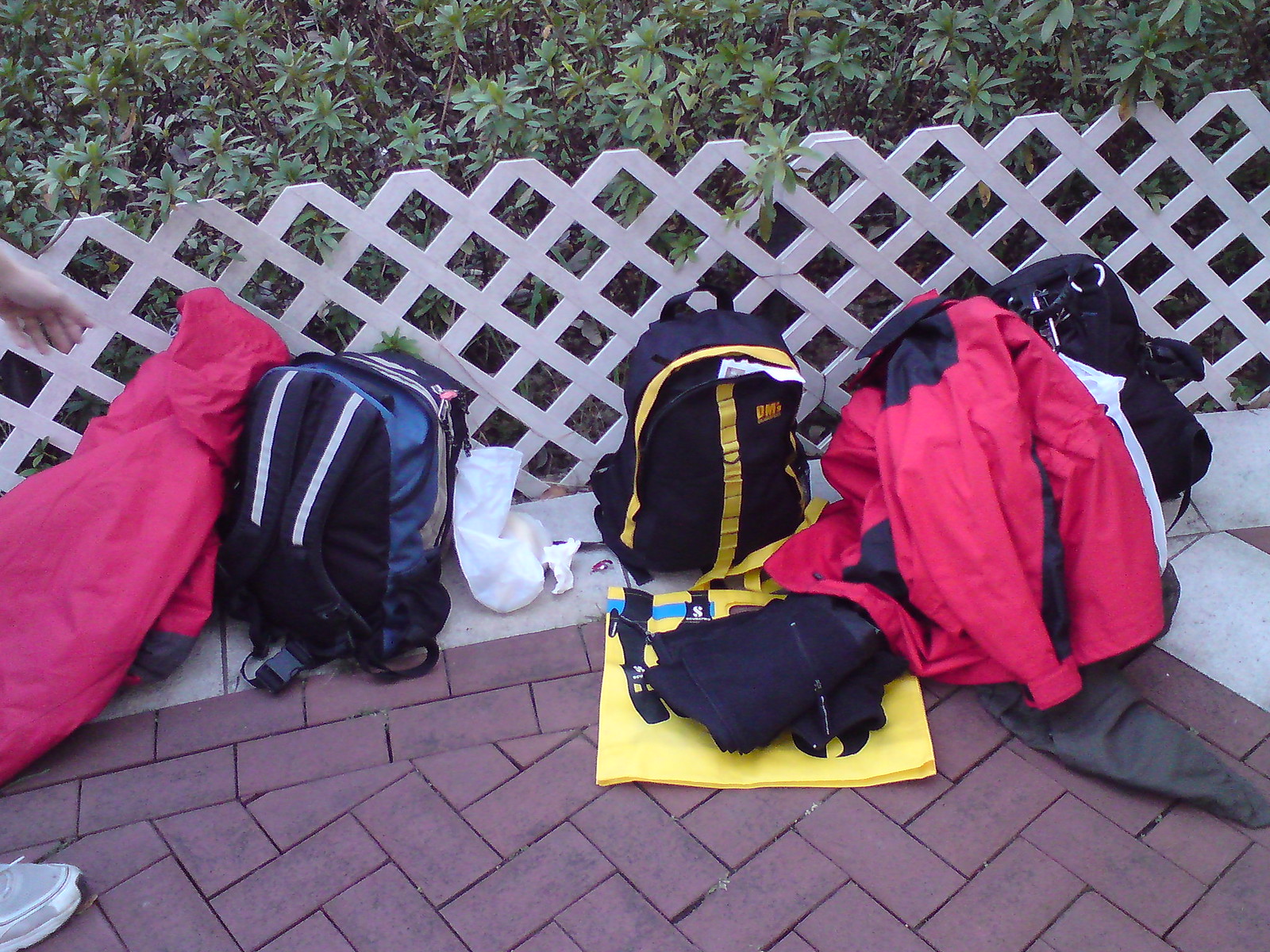The image captures a scene of travel gear organized on a red interlocking brick floor with a white border, viewed slightly from a human height angle. Against a cross-hatched white picket fence, partially covered with green bushes resembling rhododendrons, various items are neatly arranged. Prominently displayed are three backpacks: one predominantly blue with black straps and gray reflective stripes, another black with yellow stripe accents, and a third black backpack partly hidden under a red jacket. Two vibrant red coats, possibly raincoats, lie adjacent to the backpacks. Notably, a large white sock is positioned between two of the backpacks. A yellow mat hosts some of the items, and partially visible are a sneaker and a human hand reaching into the scene from the lower left corner of the photograph. The background features the stone floor and intricate plastic barriers adding depth to the composition.